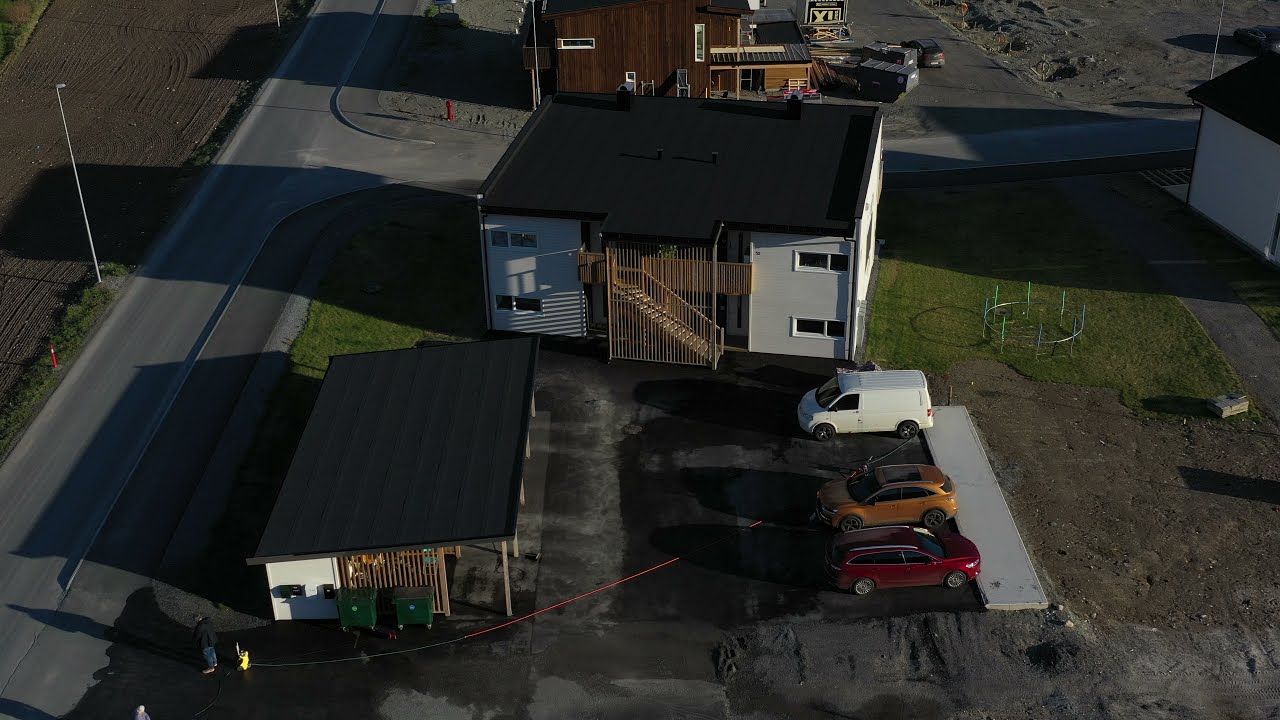This overhead photograph captures a two-story apartment building at the center, characterized by a gray exterior and a black roof. The apartment building features a total of four front-facing windows, with two on each level, flanking a central wooden staircase covered by a slatted partition. Positioned directly in front of this building in the lower left corner is another single-story structure with a dark roof which may serve as a garage or covered parking area.

To the right of this foreground structure is a clearly defined parking area where three vehicles are prominently parked: a white van, an orange metallic car, and a red car. Additionally, there appear to be more vehicles, though partially obscured, suggesting a black car and a gold car. The parking area extends horizontally across the bottom right of the image.

The left side of the image features a roadway running vertically upwards from the lower left corner towards the upper left segment, past the apartment building. Adjacent to this road is a streetlight. In the upper right corner, another building casts a dark shadow, while a separate darker wooden building can be seen toward the uppermost center. Finally, in the background, beyond the apartment building, is a small brick structure with an indeterminate sign, possibly indicating a store or post office, and a grassy yard area is visible to the right of the main building.